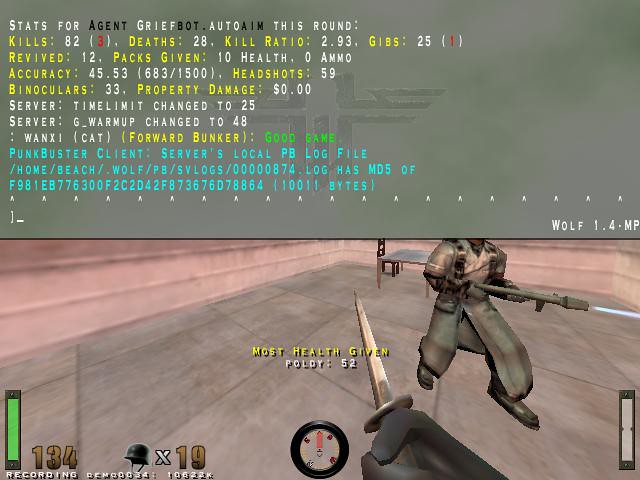This screenshot from a video game, likely played on a computer, highlights the statistics for a character named Agent Grief in a chaotic, combat-driven environment. At the top half, the screen displays a detailed stats window with the text "Stats for Agent Grief, Bot Auto, Aim This Round" in a mix of red, yellow, white, and blue fonts. Specific statistics enumerated include 82 kills (with a ranking of 3), 28 deaths, a kill ratio of 2.93, 25 Gibbs (ranked number 1), 12 revives, 10 axe given, zero health, 45.53% accuracy, 59 headshots, and binocular usage among other metrics.

In the lower half of the screenshot, the gameplay footage captures a character, partially obscured, dressed in a tan military uniform and holding a weapon on a concrete floor with concrete walls, indicating a stark, utilitarian environment. The weaponry hints at a combat scenario, likely violent given the emphasis on kills and weapon stats. Other graphical elements include a recording indicator marked with the number 134, a green rectangular bar near this text, and an icon of a helmet with the number 19, which might signify items or health packs available. The backdrop remains relatively nondescript, affirming the concrete setting but offering little indication of the game's specific location or storyline.